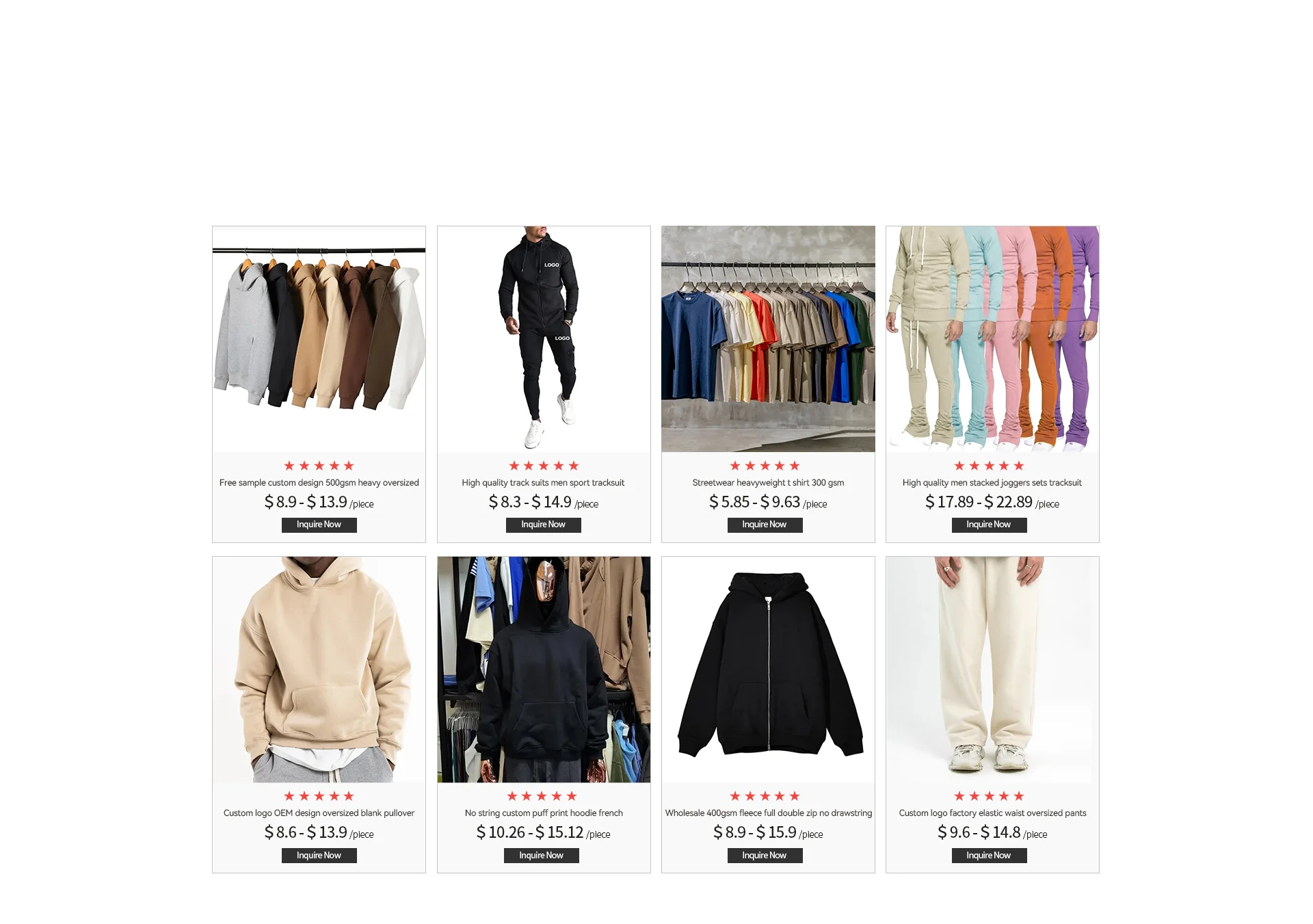Here is a detailed and cleaned-up caption for the screenshot of the Shopify example page:

---

The screenshot depicts what appears to be a Shopify example page showcasing eight distinct apparel items on sale, each offering varied selection options and price ranges, likely due to different available colors and sizes. 

1. **First Item**: A brightly displayed rack featuring seven sweaters in a spectrum of colors: gray, white, black, beige, cream, brown, and forest green.
2. **Second Item**: A man modeling a complete tracksuit paired with white tennis shoes, emphasizing comfort and athletic style.
3. **Third Item**: A collection of multi-colored t-shirts arranged on a rack, showcasing a variety of hues to choose from.
4. **Fourth Item**: An image of four individuals each wearing pajamas in different colors, suggesting cozy and diverse sleepwear options.
5. **Fifth Item**: Depicts a simple hoodie, followed by:
6. **Sixth Item**: Another alternative hoodie design, and:
7. **Seventh Item**: Yet another hoodie, each likely differing in style, color, or material.
8. **Eighth Item**: A close-up of cream-colored pants or shoes, though the focus is unclear without further detail.

Each product on this page holds a five-star rating, while the titles remain too small to decipher, implying that this could be a mock-up or illustrative example page rather than an actual store inventory.